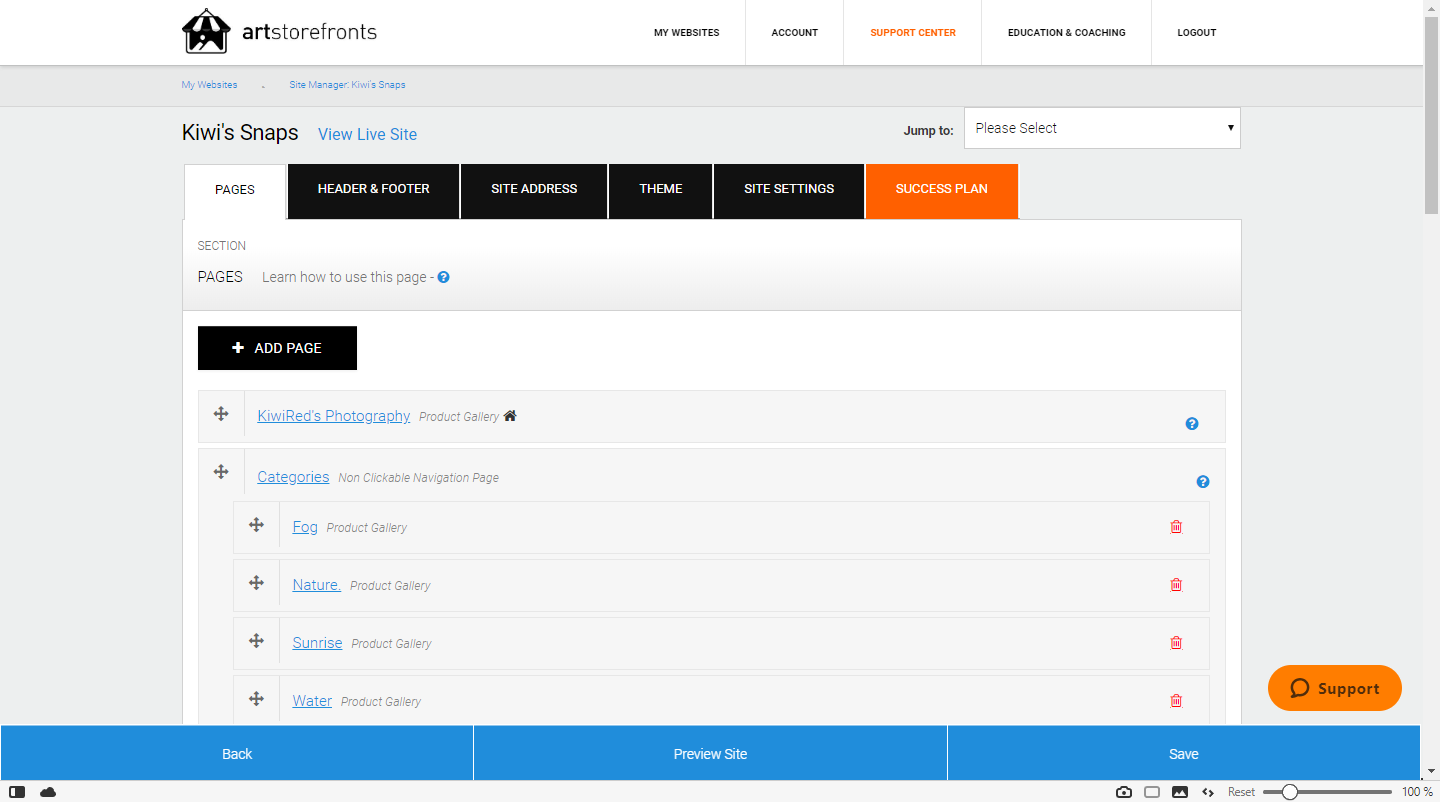A detailed screenshot of the Arts Store Fronts website displays the user interface for managing a photography website named "Kiwi Snaps." The website features a grey background with a central options box. At the top, a navigation menu includes selections for 'My Websites,' 'Account,' 'Support Centre,' 'Education and Coaching,' and 'Logout.' The 'Support Centre' option is highlighted in orange.

In the main section, the title "Kiwi Snaps" appears prominently, accompanied by options to 'View' and 'View Live Site.' Below, a menu provides management tools: 'Pages,' 'Header and Footer,' 'Site Address,' 'Theme,' 'Site Settings,' and 'Success Plan.' The 'Pages' tab is currently selected, indicating the user is managing page content.

A subheading instructs, "Learn How To Use This Page," with an adjacent blue button featuring a question mark icon for on-screen assistance. Beneath this, a black rectangle labeled 'Add Page' invites the user to create new pages.

Listed below are the current pages added by the user. "Kiwi Red's Photography," linked in blue, likely serves as the homepage. Underneath, additional pages include 'Product Gallery,' 'Little House' (designated as the home page), and 'Categories,' also linked in blue. The 'Categories' section elaborates with subcategories: Fog, Nature, Sunrise, and Water, demonstrating the site's organization of photo content.